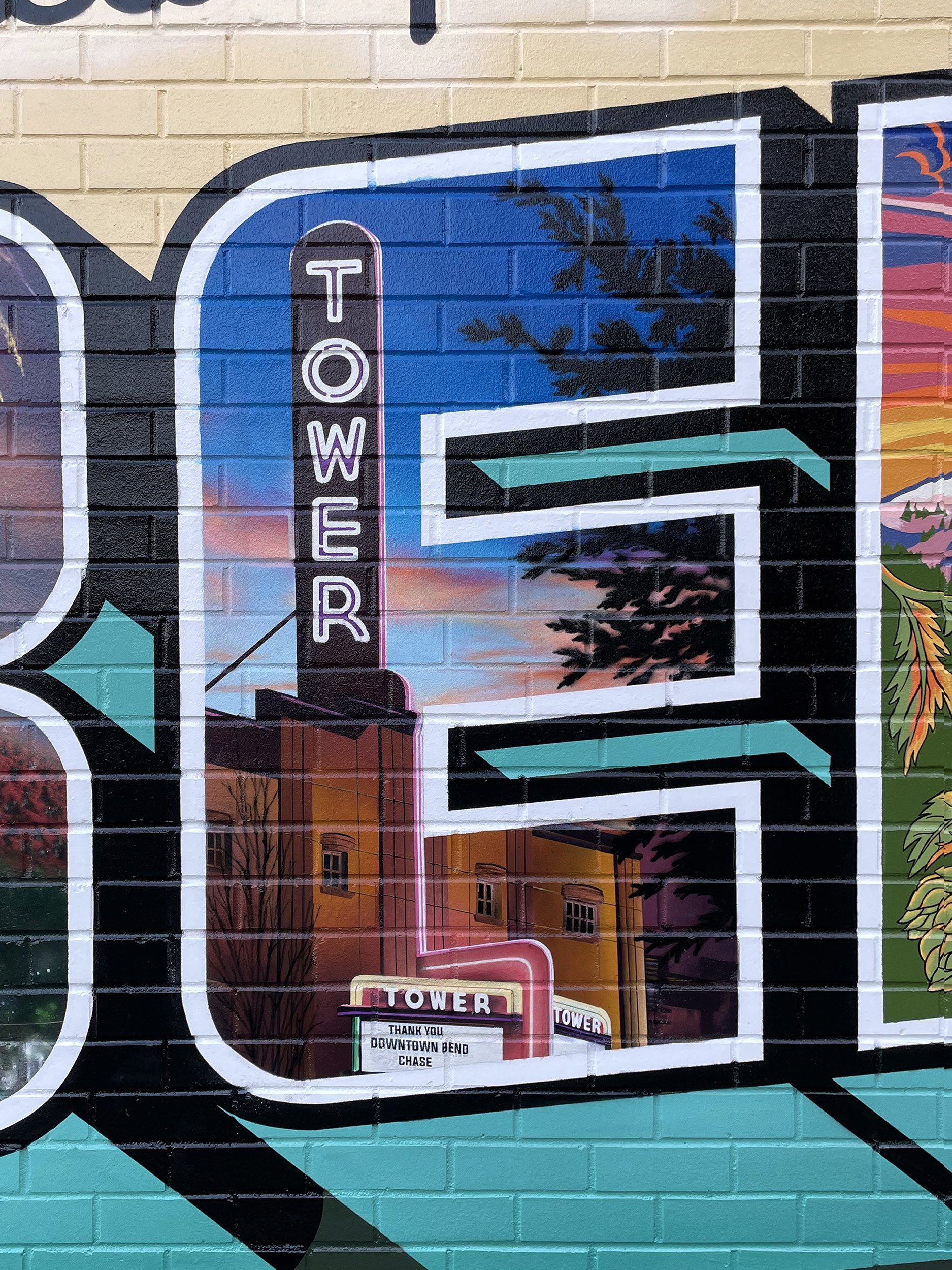The image is a detailed, zoomed-in section of a vibrant street art mural painted on an exterior brick wall. The focal point of the mural is a large, balloon-styled letter "E." Inside the "E," a realistic depiction of the Tower Theater, seemingly located in downtown Bend, takes center stage. The theater features a vintage marquee that reads "Tower Theater" with neon lights and a tall, vertical sign that spells out "Tower." The marquee also has a welcoming message that says, "Thank you, downtown Bend" and "Chase," which could refer to names of shows or sponsors. Surrounding the theater, the mural artist has painted a beautiful twilight sky, blending hues of pink and dark blue to evoke a sunset. Additionally, some trees frame the right side of the "E," adding to the mural's depth and liveliness.